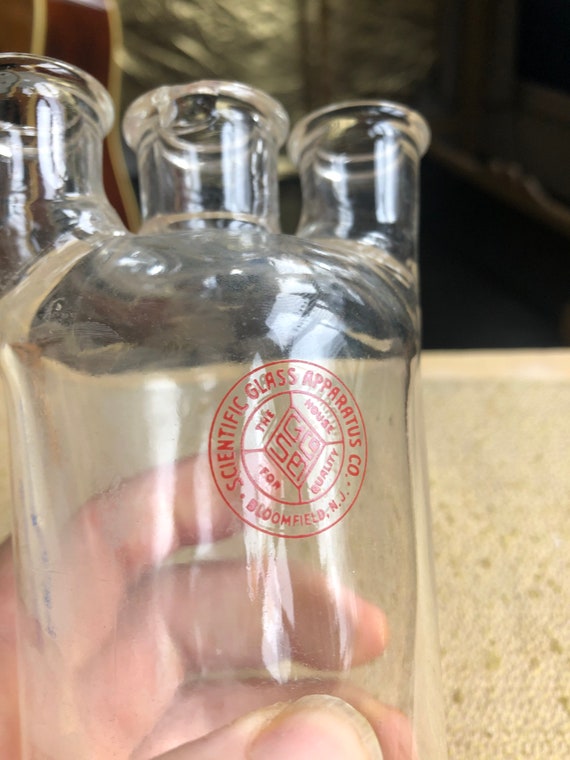In this detailed photograph, a left hand is prominently featured, holding a glass apparatus designed for scientific use. The hand, positioned on a beige table, grasps the glass with the thumb and the first two fingers. The glass apparatus appears large and slightly heart-shaped, with three openings at the top likely intended for connecting hoses or pipes. The apparatus is empty, accentuating its transparency, through which the person’s fingers are visible.

The apparatus displays a circular red logo with clear lettering that reads, “Scientific Glass Apparatus Company, Bloomfield, New Jersey.” In the center of this logo, additional text reads, “The House for Quality,” accompanied by some squiggly line symbols, and possibly the letters "GS," slightly obscured by glare. The background includes a silver object and a red object, adding subtle contrast to the image. The top half of the background transitions from black to light gray, enhancing the visibility of the glass apparatus.